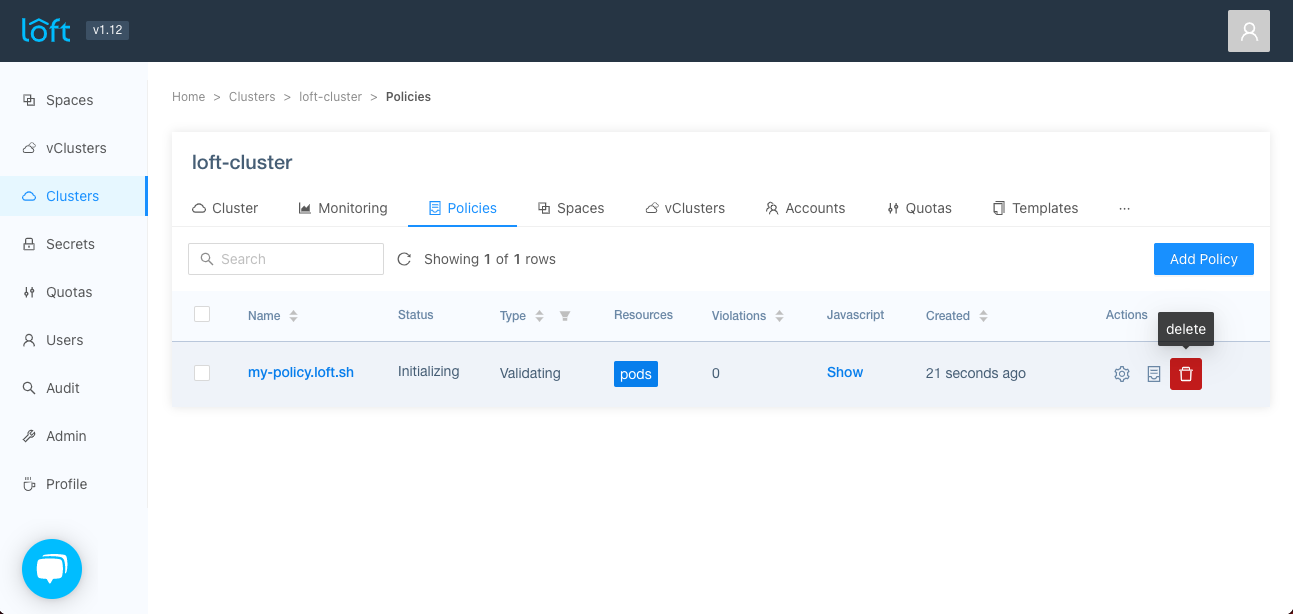This screenshot features a user interface predominantly characterized by a white background with a sleek black border at the top. In the top-left corner, the word "loft" is prominently displayed, while in the top-right corner, a gray square housing a generic profile silhouette image can be seen. The interface has a vertical sidebar on the left, presenting a list of small icons accompanied by explanatory text. This list includes: Spaces, vClusters, Clusters (highlighted), Secrets, Quotas, Users, Audit, Admin, and Profile. Below these items, a blue circle with a speech bubble icon is visible.

In the main section of the page, navigation breadcrumbs guide the user, starting with "Home," followed by a small arrow, then "Clusters," another small arrow, "Loft Cluster," another arrow, and finally "Policies" which is highlighted. Below the breadcrumbs, a bold header reads "Loft-Cluster," accompanied by a cloud image and the label "Cluster." 

Tabbed navigation is horizontal across this section. The tabs, in order, are: Cluster, Monitoring, Policies (highlighted in blue and underlined), Spaces, vClusters, Accounts, Quotas, and Templates. 

On the left side beneath the tabs, there is a search box with the word "Search" pre-entered. The page informs the user it is "Showing 1 of 1 rows." A table below this notification displays several columns with headers: Name, Status, Type, Resources, Violations, Javascript, Created, and Actions.